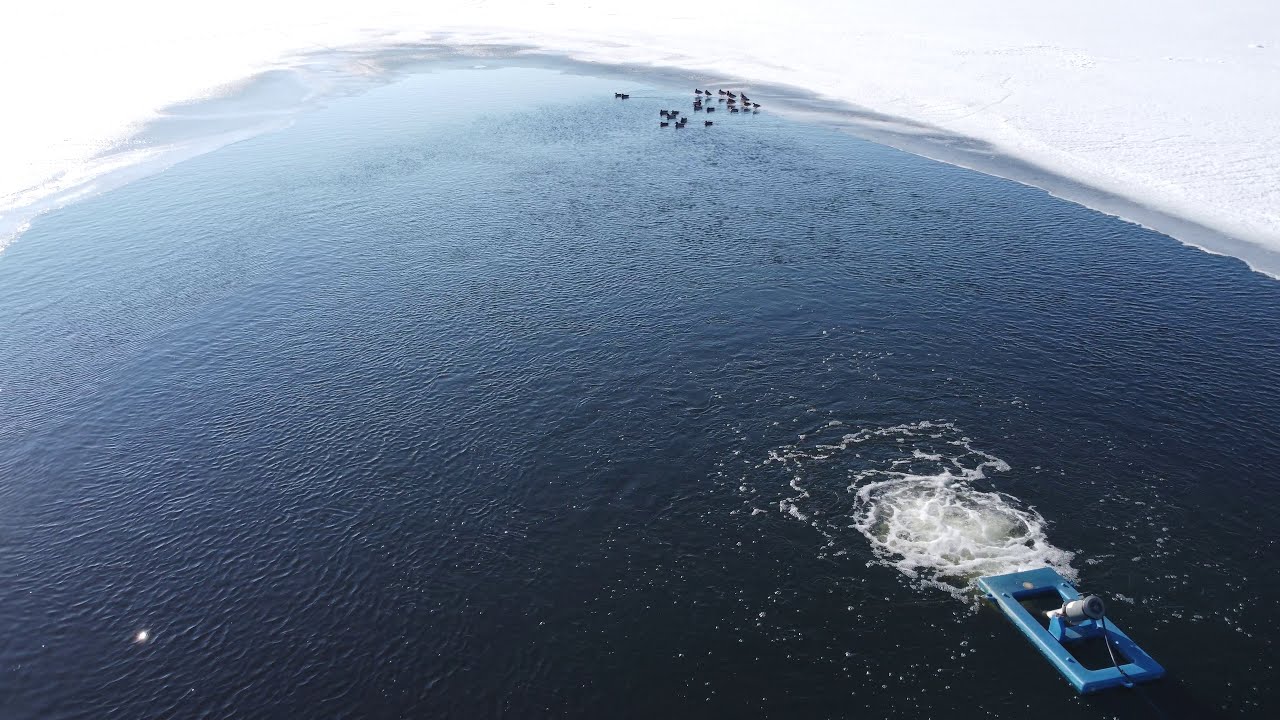This high-angle, possibly drone-captured image depicts a vibrant blue body of water encircled by sprawling sheets of ice and snow, likely indicating a frozen lake or a section of the frozen ocean, implying perhaps an Arctic or Antarctic setting. Central to the image is a small, box-like blue structure floating on the water, outfitted with a cylindrical device that extends downward, emitting bubbles. This setup seems to be an oxygenating pump or filtration device, complete with a blue frame and a prominent black power cable, designed to circulate and aerate the water. 

Adjacent to this scene, a group of water birds, possibly ducks or penguins, are gathered at the icy edge of the water, hinting that the water might be shallow at this end but deepens further out. The water itself is a rich blue, reflecting the sunlight, providing a stark contrast to the surrounding icy expanse. The image's fisheye effect slightly distorts the scene, giving it a wrap-around appearance and enhancing the surreal, almost other-worldly feel of this icy, aquatic environment.